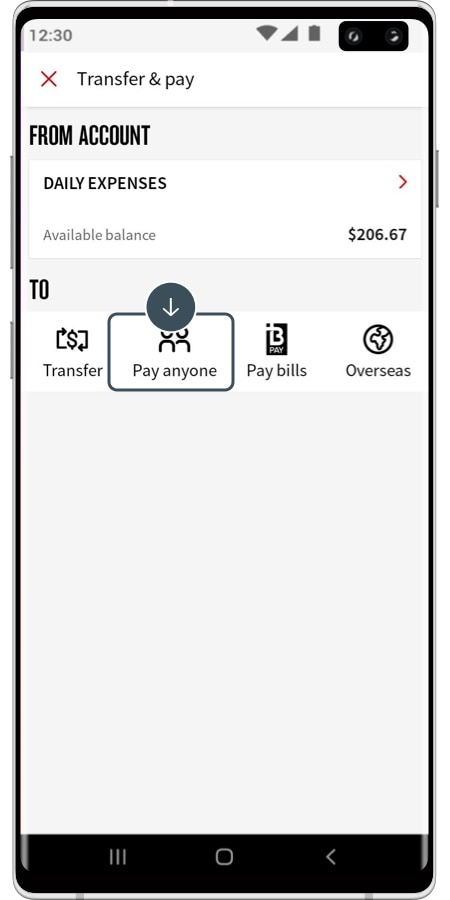The image depicts a smartphone with visible bezels and side buttons, including the power button and volume controls. The screen displays a financial app interface, detailing a money transfer. The status bar at the top shows the time as 12:30 and a full battery at 100%. The screen features a white background with a top banner reading "Transfer and Pay," accompanied by a red 'X' icon on the far left. Below the banner, the text indicates the transaction is from the account labeled "Daily Expenses," with an available balance of $2,267. The main focus of the screen is the transfer interface, where "Pay Anyone" is highlighted, suggesting a transfer function. Surrounding this highlighted option are three other buttons: "Transfer" on the left, "Pay Bills" on the right, and "Overseas" further to the right. The overall display gives a clear depiction of a financially-focused app designed to facilitate various transactions, suggesting the user is about to initiate a transfer from the Daily Expenses account to pay an individual.